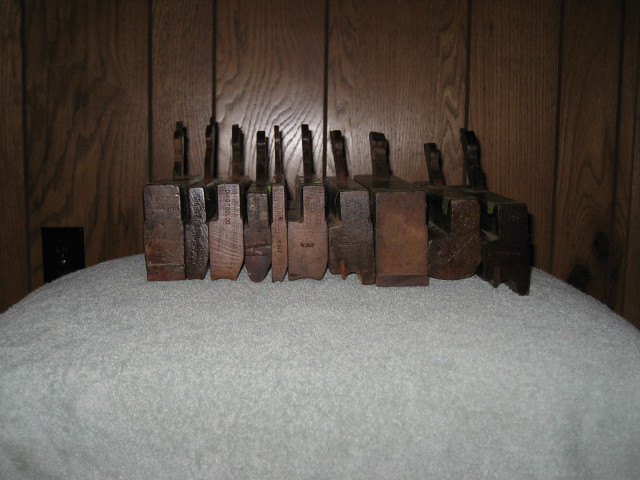The color photograph captures a collection of vintage wooden molding planes, used by craftsmen and carpenters for creating various molding designs. These antique tools, exhibiting rounded edges and rounded corners from extensive use, are neatly arranged in a row on a large light gray cushion or blanket. The background consists of dark wooden paneling, providing a striking contrast to the planes. Each plane features a vertical grab handle protruding from the back and some display profile images indicating the molding shapes they create. While the photograph offers a detailed view of the planes’ different angles and designs, it lacks any writing, people, animals, or other objects, focusing solely on these historical woodworking implements.